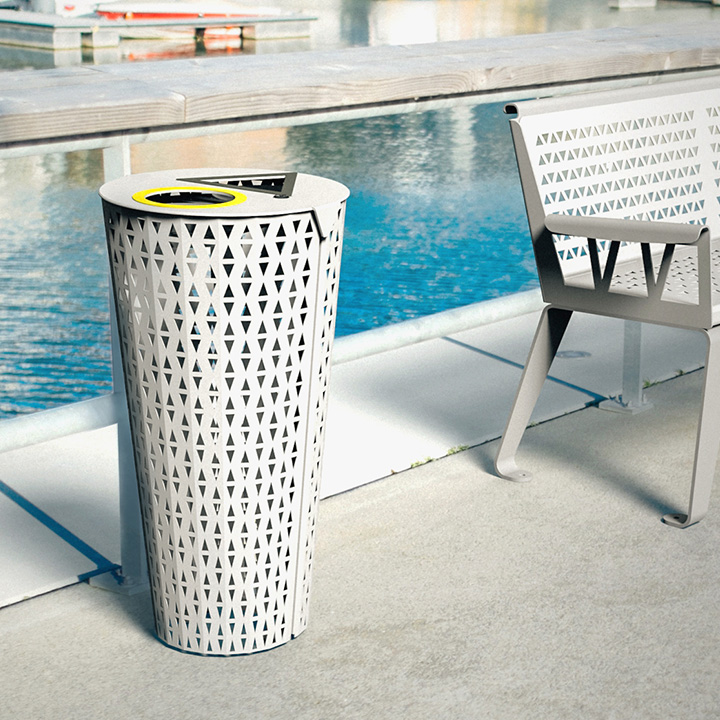This photograph captures a serene scene by what appears to be a narrow lap pool or water feature. The foreground is a concrete walkway, adorned with large white tiles grouted in blue. Prominently featured is a tall, slender metal trash can, painted white with an intricate pattern of triangular cutouts. These cutouts are arranged in various end-to-end and tip-to-tip configurations, creating a visually appealing design. The trash can widens slightly at the top, which is distinguished by two openings: a small yellow-rimmed circle and a black-rimmed triangle, likely indicating sorting for recycling and garbage.

Adjacent to the trash can, approximately two and a half feet to the left, is a matching white metal bench. The bench echoes the trash can’s retro 1960s aesthetic with the same triangular cutout pattern and features a triangle-shaped armrest. Behind these items is a narrow, inviting pool with a striking aqua blue hue. Beyond the pool, there's a wooden bench, made from unstained and slightly faded wood, sitting atop what may be a dock or continuation of the pool area. The combination of the modern, patterned metalwork set against the tranquil water and simple wooden elements creates a harmonious blend of design and nature.